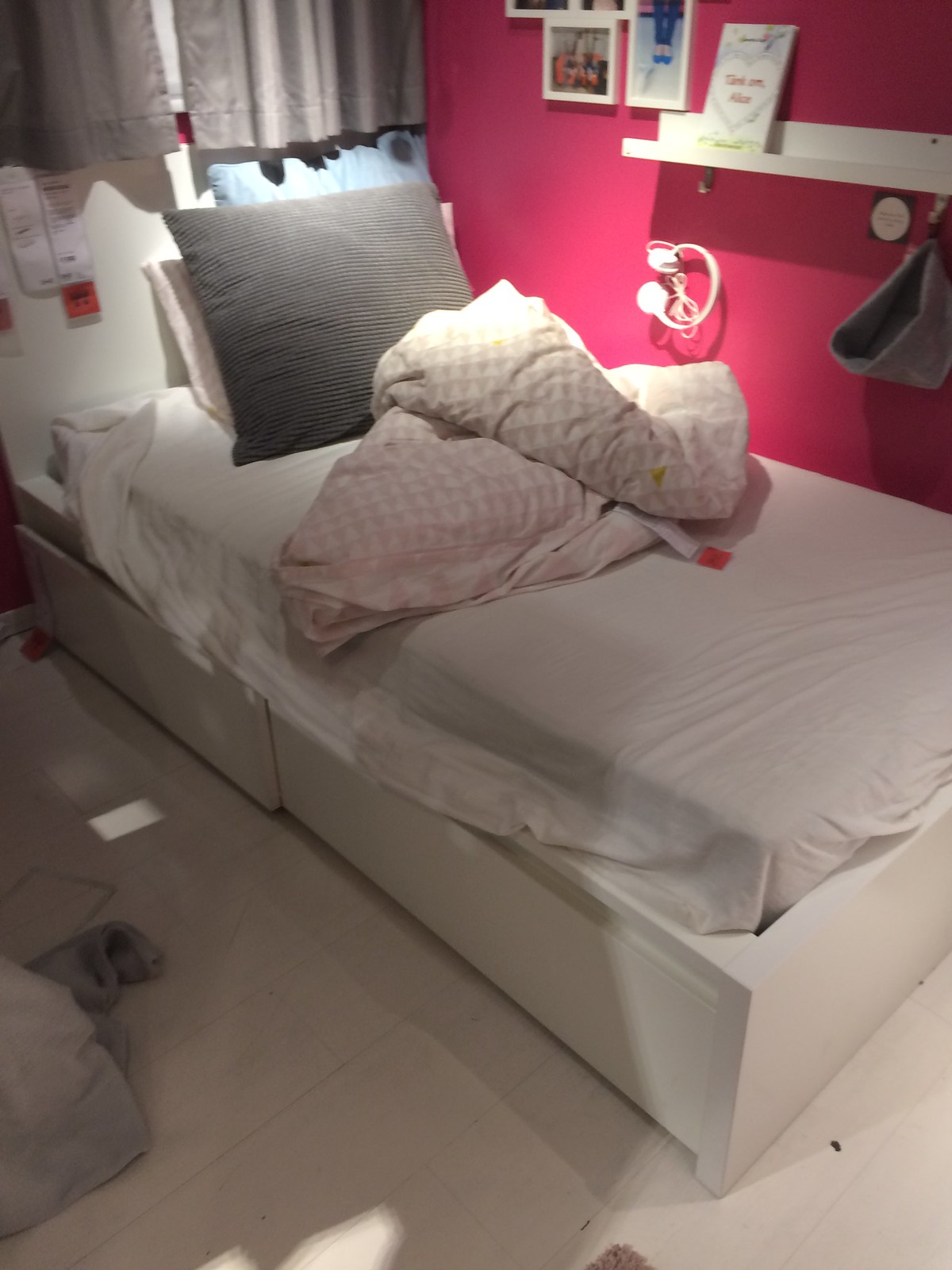This is a detailed photograph of an IKEA-styled bedroom, presented as part of a showroom display. The main feature is a twin-sized, multifunctional box bed with white pull-out drawers at the base, showcased at a diagonal angle. Draped over the bed is a ruffled duvet with a pattern of white and light pink triangles, casually folded over itself. The bed is adorned with three pillows: a light blue one, a gray striped one, and a white one underneath. The bed is placed against a deep hot pink or fuchsia wall, which is partly covered by gray curtains. 

Additional details in the room include a white shelf mounted on the pink wall, from which a pair of white headphones hangs. Below the shelf, there's a small gray bag that appears to be for storage. The wall also features two photographs and the signature IKEA product tags displaying information about the furniture pieces and their locations in the store. The floor is made of white or cream tiles, and there are noticeable shadows cast, suggesting natural light streaming in from an unseen source. The overall setup gives a balanced blend of function and style, characteristic of an IKEA bedroom arrangement.